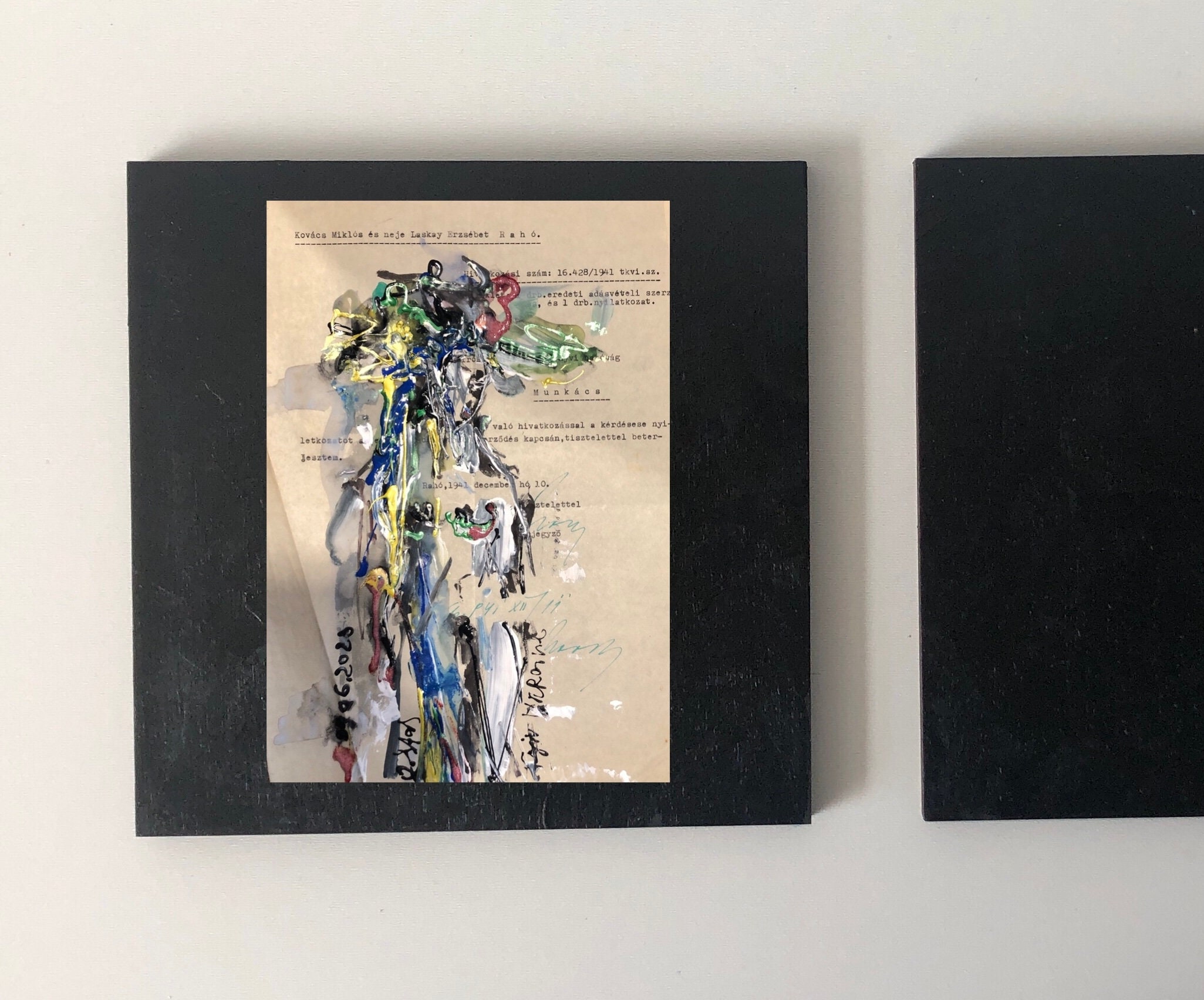This photograph captures an artwork mounted on a white wall, featuring two black frames, although the one on the right is partially out of view. In focus is the left frame, which holds a semi-three-dimensional collage set against a black background. The centerpiece of this collage is a slightly yellowed, vintage piece of paper, adorned with both printed and handwritten text. While the precise content of the text is not entirely legible, portions of it appear to be in a foreign language, with strings of letters like "Kovace" and "62025" scattered among the script. The artwork is richly textured, featuring an abstract burst of vibrant colors—red, blue, green, yellow, rose, white, and gray—sprawled across the paper. These paint blobs and strokes form a chaotic yet visually engaging composition. The colors are most densely packed toward the top of the paper, creating a semblance of a mountain or an explosion, and then spread more sporadically toward the middle and bottom. The colorful drips and smears suggest a creative frenzy, with some hints of stylized forms or patterns etched amid the vibrant chaos.